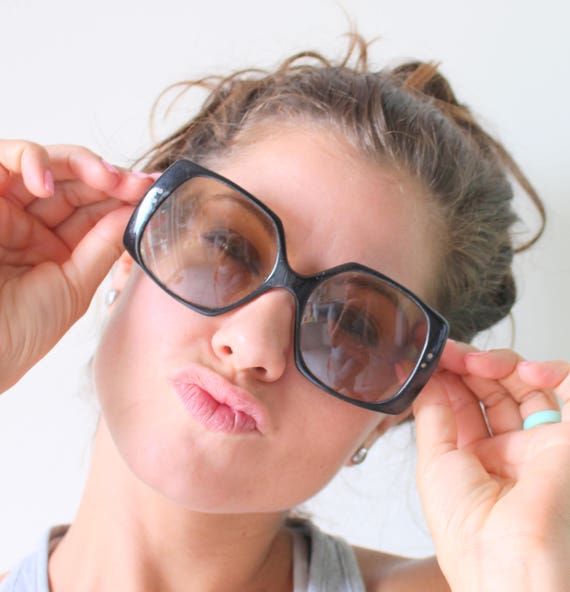The image is a color photograph in a square format, showcasing a young Caucasian woman in her 20s or 30s. She's posing with oversized, squarish sunglasses featuring smoky lenses and thick, black rims. Her skin has a light pink hue, and she has brown hair tied behind her head. The woman is making a playful pouty, kiss-like face often referred to as "duck lips." Both of her hands are visible, holding the sunglasses on either side of her head. Silvery, metallic reflective earrings dangle from her ears, and a ring adorns the ring finger of her left hand. She appears to be wearing a gray tank top or halter top, though only her neck and a small portion of her shoulder are visible. The background is a light gray, enhancing the realistic and product photography aspects of the image.